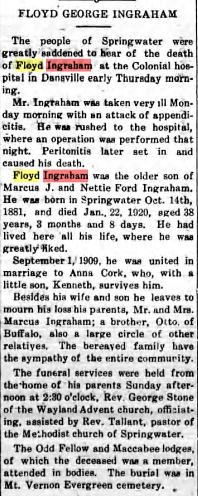The image is a vertically oriented newspaper obituary highlighted with the name "Floyd Ingraham" in two instances. The name "Floyd" is highlighted in yellow, while "Ingraham" is highlighted in red. The text states that Floyd George Ingraham, the elder son of Marcus J. and Nettie Ford Ingraham, was born in Springwater on October 14, 1881, and died at the age of 38 on January 22, 1920, at the Colonial Hospital in Danville following complications from an appendicitis operation. He was beloved in his community and lived in Springwater his entire life. Floyd married Anna Cork on September 1, 1909, and they had a son named Kenneth. Besides his wife and son, Floyd is mourned by his parents, a brother named Otto from Buffalo, and a large circle of other relatives. His funeral was held at his parents' home on a Sunday afternoon, with services conducted by Reverend George Stone of the Wayland Advent Church, assisted by Reverend Talent of the Methodist Church of Springwater, along with the Odd Fellow and Maccabee lodges. Burial took place at Mount Vernon Evergreen Cemetery. The community extended their heartfelt sympathies to the grieving family.